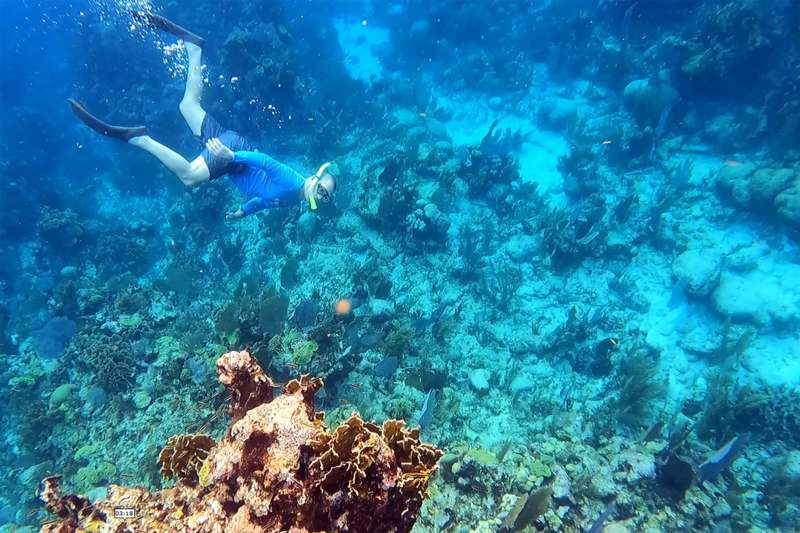This underwater photograph in landscape orientation captures a snorkeler descending into a world of blue hues. Clad in a blue t-shirt, black half-pants, and black fins, he navigates through the tranquil waters with a yellow snorkel and dark-rimmed goggles. The snorkeler is positioned in the upper left corner, swimming towards the center, with bubbles rising from his snorkel. The scene is bathed in varying shades of blue, from the light above to the deeper tones below. On the floor of this aquatic environment lies a diverse array of rocks and water plants, predominantly blue, but accented by a striking brown coral reef in the lower left corner, which contrasts sharply against the blue backdrop. This particular piece of coral appears tan and beige-ish and draws the snorkeler's attention. Additionally, a small tab marked "18" is visible in the photo, identifying the print. The overall composition beautifully captures the serene yet vibrant underwater ecosystem, highlighting the interaction of light, colors, and marine life.